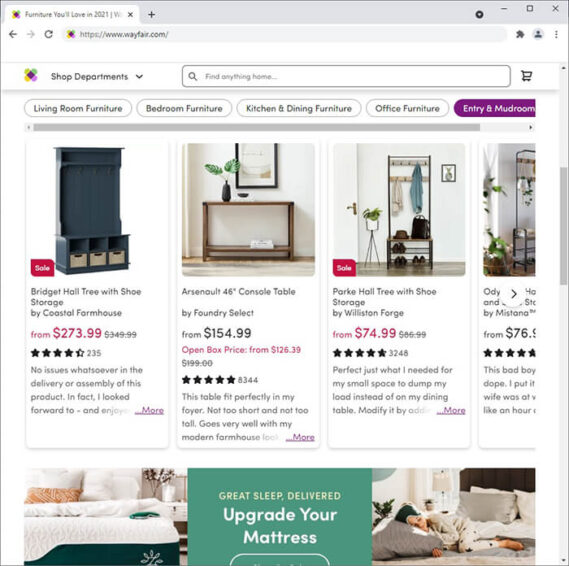This is a screenshot of a web page from a computer monitor showing the Wayfair.com website. The browser's address bar displays the Wayfair URL, and directly beneath it is the site's header. The header features the Wayfair logo, followed by a drop-down menu labeled "Shop Departments." Next to the drop-down is a search bar with placeholder text that reads "Find anything home," and to the right of that is a shopping cart icon.

Below the main navigation, there are category tabs for various types of furniture: Living Room Furniture, Bedroom Furniture, Kitchen and Dining Room Furniture, Office Furniture, and Entry & Mudroom Furniture. The current category displayed is "Entry & Mudroom."

The first product listed is a shoe storage cabinet priced at $273.99, discounted from $349.00. It has received an average rating of 4.5 stars out of 5, based on 235 reviews. The second product is a 46-inch console table, starting at $154.99, with a perfect 5-star rating from 8,344 reviews. The third item is a hall tree with shoe storage, priced at $74.99, and it boasts a 4.5-star rating from 3,248 reviews. Another hall tree is partially visible but cut off from the view.

Below the listed products, there is an advertisement promoting mattresses with the slogan "Great Sleep Delivered, Upgrade Your Mattress." The ad features images of a bed on the left side and a woman lying on another bed on the right side, dressed in full pajama pants and top.